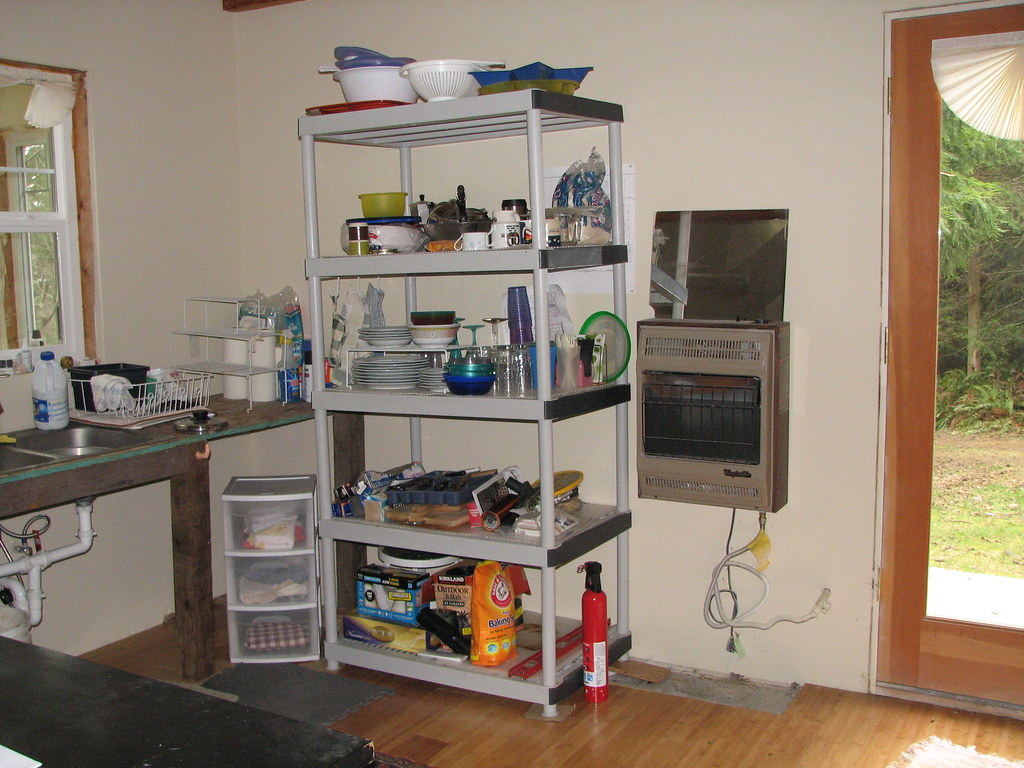In an indoor kitchen, a wooden floor extends across the room. Dominating the center is a white, five-tiered shelving unit filled with various kitchen items – dishes, plates, cups, and a drainage bin at the top. A recognizable box of Arm & Hammer sits on the bottom shelf, beside a red fire extinguisher. To the left of the shelving unit stands a three-drawer plastic organizer. The backdrop features a clean, white wall, and a window is visible on the left side, letting in natural light. White piping runs along the bottom left, and a fan hangs from the top right, providing ventilation. Towards the back, there is a large appliance that could be an oven or an air conditioning unit. Outside the window, a green backyard with trees offers a refreshing view, adding an element of tranquility to the functional, tidy kitchen space.